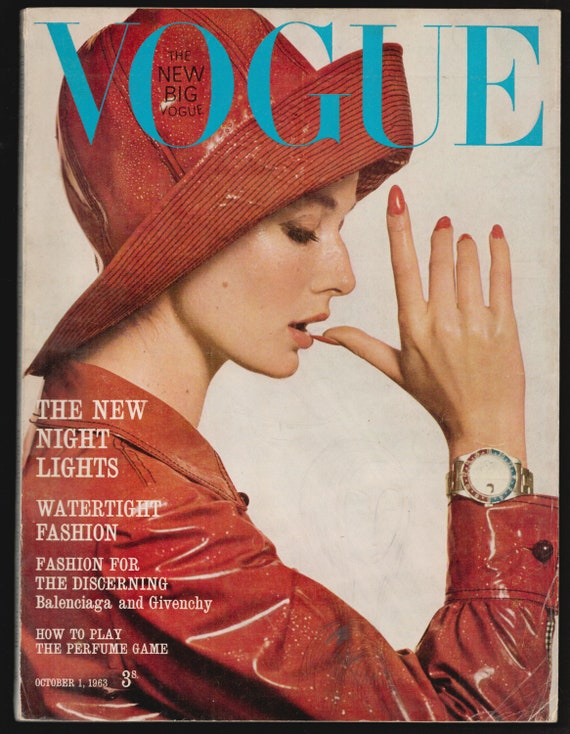This vintage Vogue magazine cover, dated October 1, 1963, is slightly taller than it is wide and features a striking black frame. Dominating the top in large, bold blue letters is the iconic "Vogue" logo. The cover stars a fashionable model, poised to the side, donning a glossy red raincoat paired with a matching rain hat, its brim stylishly flipped upwards at the front.

The model's eyes are either closed or looking downwards, and she raises her hand with her thumb and bright red-orange polished nail resting on her bottom lip, exuding an aura of sophisticated contemplation. A sizable watch adorns her wrist, adding to her chic ensemble.

Overlaying the image in white letters are various intriguing articles inside this issue, including "The New Nightlights," and "Watertight Fashion," suggesting an exploration of rain-ready haute couture. Additionally, it promises insights into "Fashion for the Discerning: Balenciaga and Givenchy," and advice on "How to Play the Perfume Game." At the bottom left, the price is listed as $3.80, with a large white "3" and a small "S" indicating this is likely the third issue of the year. Despite its age, the cover maintains a timeless elegance.